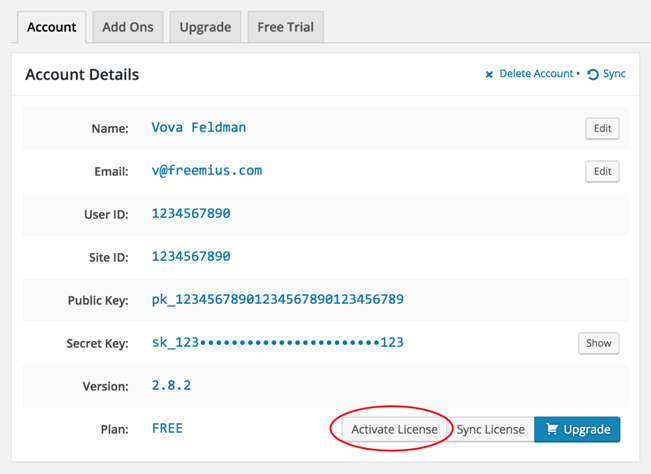**Descriptive Caption:**

This is a detailed view of the "Account" page on a user's profile within a website. The page is organized with several navigational tabs at the top including "Account" (currently active), "Add-ons," "Upgrade," and "Free Trial." 

Below the tabs, a series of account details are listed vertically, starting with the user's name, Vova Feldman, and followed by their email address, which utilizes a freeius.com domain. The unique User ID and Site ID are both displayed as "123456789-0." 

Further down, the user's Public Key is labeled as "PK_123456789-0_123456789-0" and the Secret Key reads as "SK_123...123," with the middle portion obscured by dots for security. 

The system version is noted as "Persian 2.8.1," and it indicates that the user's plan is currently "Free." There is a prominent option circled in red labeled "Activate License," followed by a "Sync License" button. Additionally, a shopping cart icon is visible, offering an upgrade path, while various edit options are located to the right of the account details section. These options allow the user to delete their account, sync it, and make edits to their name and email. The Secret Key can also be revealed upon request.

At the bottom, a blue box highlights another opportunity to purchase an upgrade, emphasizing that the user is on the free version of the service.